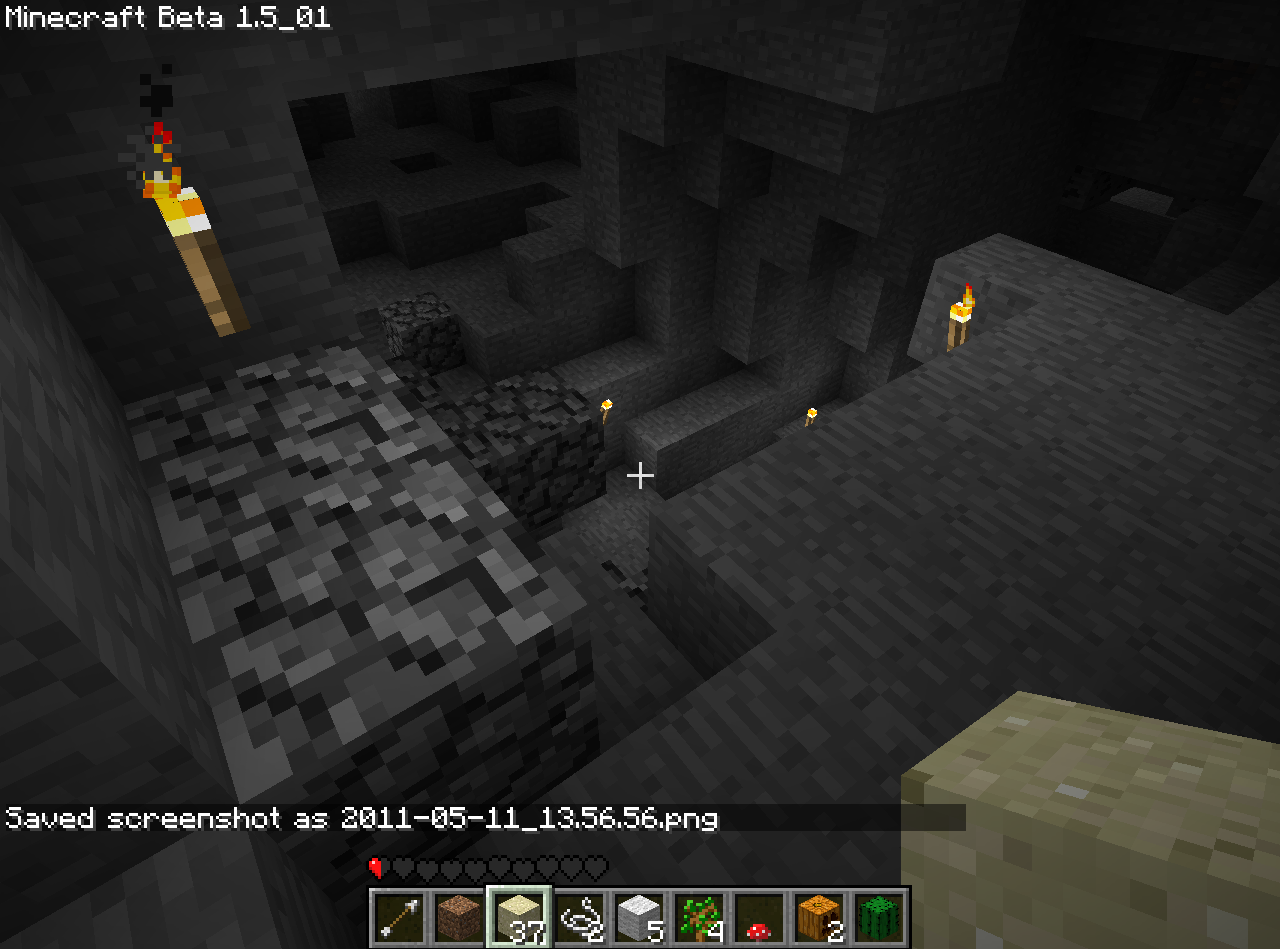This is a detailed screenshot from the computer game Minecraft, specifically from the Beta 1.5_01 version, as indicated by the white overlay text in the upper left corner. The bottom of the image also features white text reading "saved screenshot as 2011-05-11_13.56.56.png." The scene is mostly dark, depicting an underground dungeon-like space with gray, blocky walls and flooring. A pixelated torch, characterized by a brown handle and a squared-off flame, is mounted on the upper left corner of the space. The center of the screenshot reveals steps leading downwards, suggesting a labyrinthine structure. In the lower right corner, there is a block that appears to be tan and brown, and possibly a protruding dark green wall. Additionally, the bottom of the image displays an inventory overlay with seven squares, the third from the right being highlighted. This contributes to the overall mystical and adventurous vibe of the game.